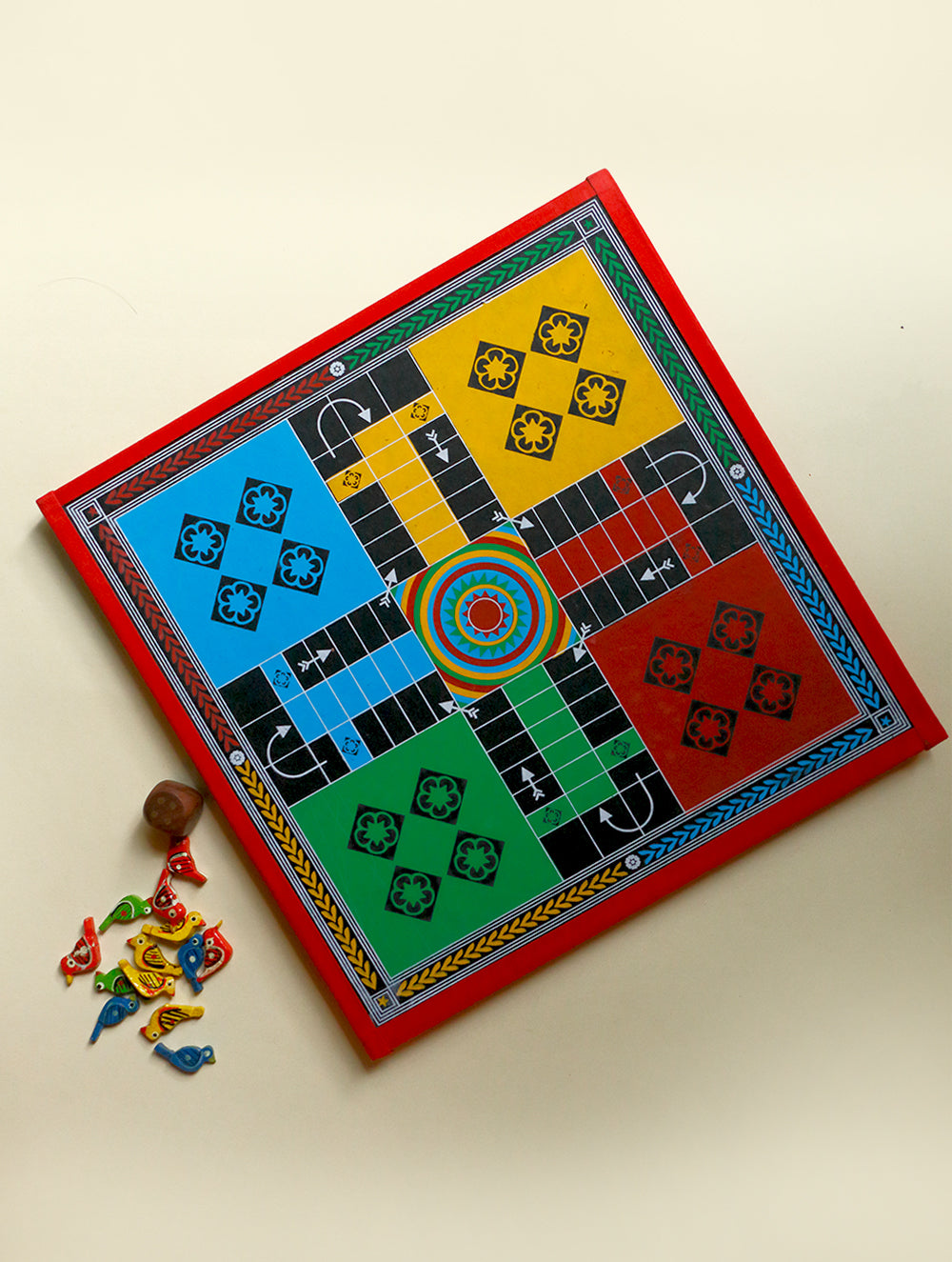This image depicts a brightly colored, square game board reminiscent of games like Parcheesi or Sari. The board is bordered in red and is divided into four quadrants: blue, green, yellow, and red, each with a corresponding colored square in its corner. The central area of the board features a multicolored mosaic of circles in a cross pattern, with pathways composed of small rectangles of dark blue and each player’s colors, leading towards the center. Lying off to the side are the game pieces, which take the shape of small birds in red, yellow, blue, and green. Adjacent to the board, there is a brown six-sided die showing the number four. The quilt-like design of the game board includes various colorful arrows and patterns that guide players in a structured manner, emphasizing the game's dynamic and engaging aesthetic.